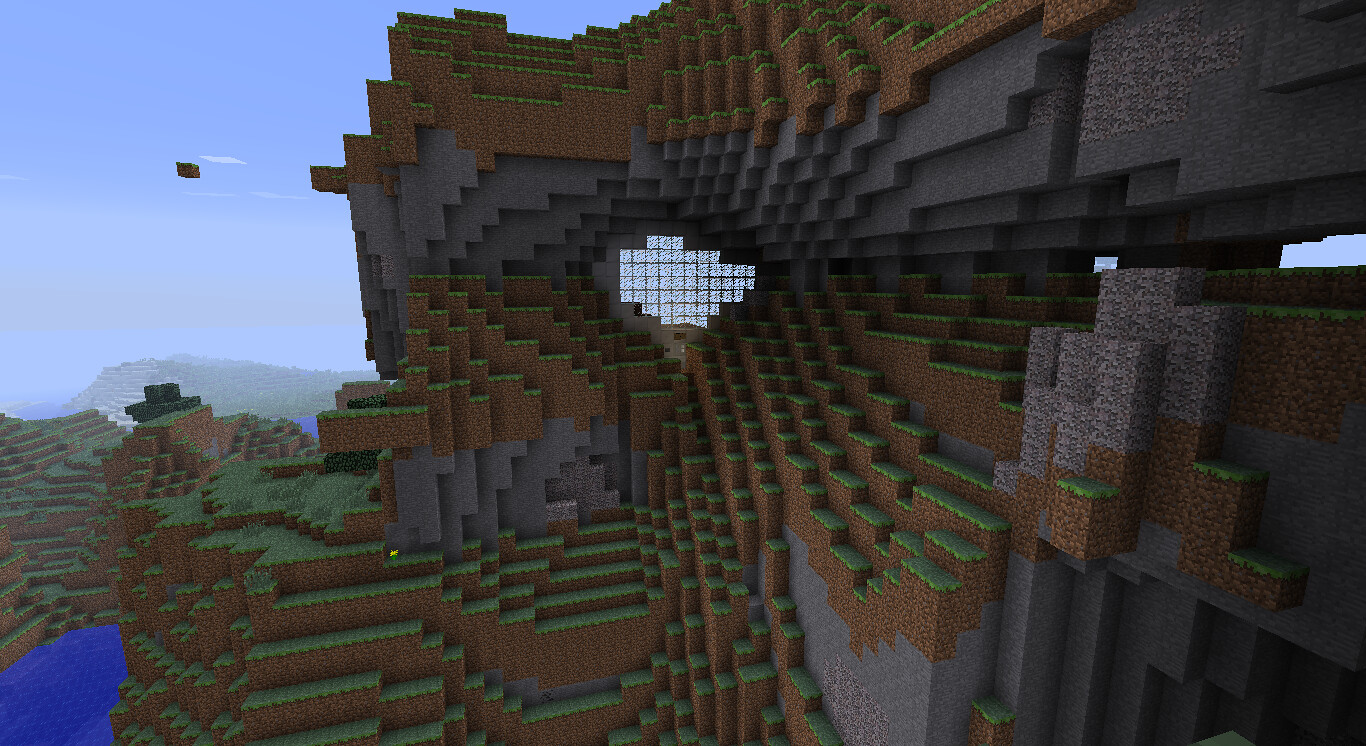This detailed screenshot from a computer-generated video game, resembling a digital Lego world, showcases a complex landscape built with interlocking bricks. Predominantly gray and brown, the structures are neatly stacked, creating a multi-leveled terrain. Green-topped bricks simulate grass or moss, emphasizing the impression of a natural landscape. Central to the image is a distinctive window made of square glass panes, surrounded by these bricks. To the right, additional windows are visible. The background reveals distant mountains, also constructed from similar bricks, enhancing the scene's depth. In the lower left corner, a closer view of mountainous structures is seen alongside a lake. Unique features like a square box floating in the blue sky, detailed with small white clouds, and what seems to be a hat on one of the brick formations, add whimsical elements to the setting. The scene portrays a virtual environment inviting creative, structure-building gameplay with a vivid, textured landscape.